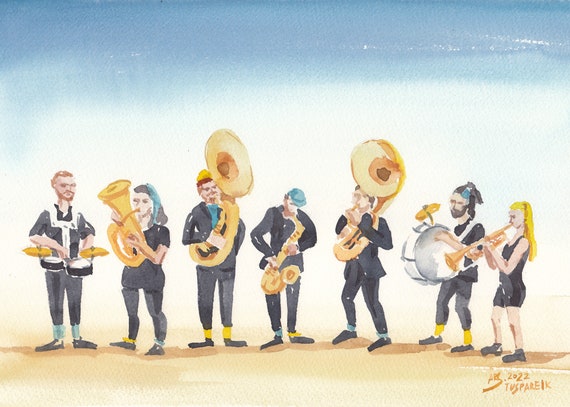This image is a detailed drawing of seven musicians playing a variety of instruments on a beach, under a blue sky that fades into white, suggesting a cloudy area. The first man on the left is playing the drums, dressed in a black and white outfit, black shoes, and blue socks. Next to him, a woman with blue streaks in her hair is playing a tuba. Moving right, there is a man playing another large instrument, possibly a trombone. The man next to him is playing a saxophone. Another man follows, also playing a large instrument, likely another trombone. To his right, another man is playing the drums. Finally, a woman at the far right is playing a trumpet. All the musicians are wearing predominantly black attire, with variations including long pants, crop pants, and shorts, suggesting either uniformity or coordinated outfits. The scene is set with the musicians standing on sand, reinforcing the beach setting. The artist's signature, "TUSPAREIK," and the year "2022" are inscribed in the lower right-hand corner of the image.